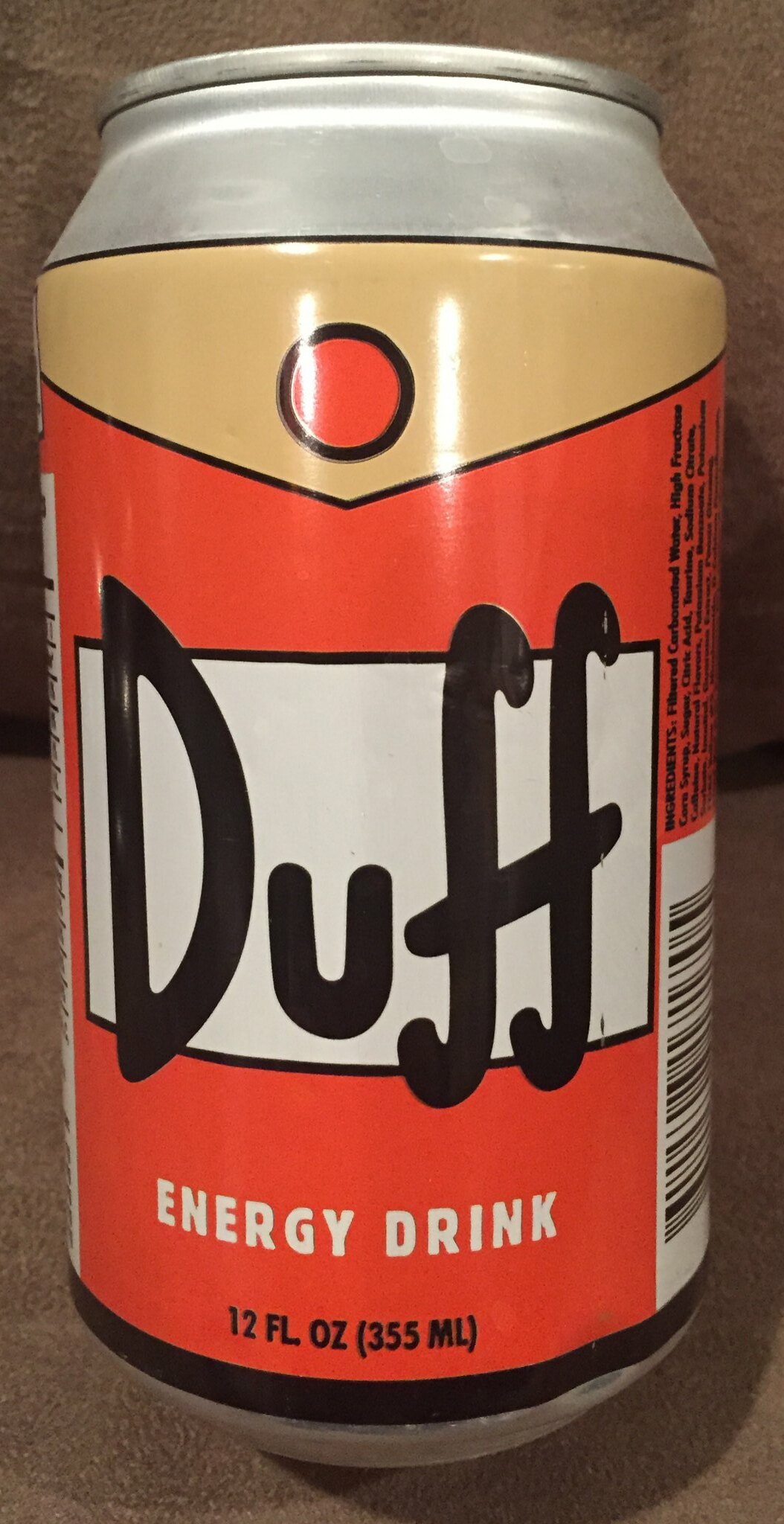The image captures a close-up of a 12-ounce aluminum can of Duff Energy Drink. The can features a bold design with a dominating bright orange color and cream-colored detailing at the top, accentuated by an angular, V-shaped triangle that contains an orange dot. The central label consists of a large white rectangle with a black border, prominently displaying the word "Duff" (D-U-F-F) in black, with the tops and bottoms of the letters extending slightly beyond the white rectangle into the orange background. Below this, "Energy Drink" is written in white lettering. The right side of the can partially reveals a black-on-white barcode and some black text listing the ingredients. The can is resting on a surface that could be a cream-colored linoleum table or carpet, with a room-light reflection visible on its metallic surface. The background appears to be a textured, medium to dark brown leather or burlap-like wallpaper, adding a rugged feel to the scene. The can casts a shadow on the supporting surface, enhancing the overall depth of the image.